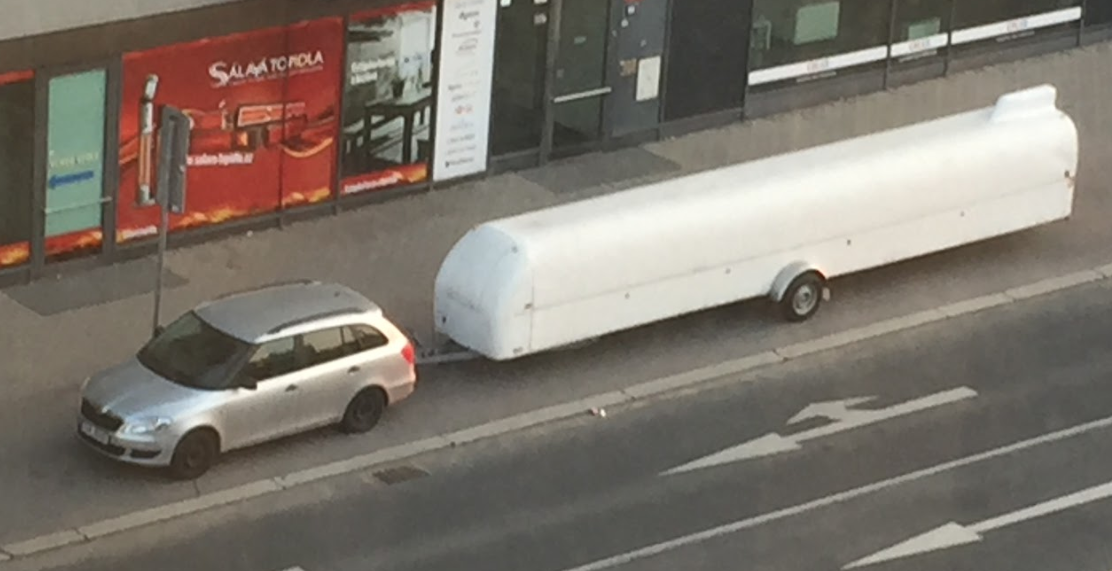In the image, a compact car is remarkably towing an extremely long white trailer, which starkly contrasts its own size. The trailer, at least three to four times longer than the car itself, features a notable fin area at its rear. Only a single set of wheels, positioned centrally on the trailer, supports the entire apparatus, suggesting an under-engineered design choice. This setup becomes even more intriguing considering the complexities of maneuvering such an elongated load through urban environments, where tight and congested corners are a common challenge. Unlike specialized vehicles like fire trucks equipped with a rear driver for efficient cornering, this trailer lacks maneuverable tires, intensifying the difficulty of navigating it through city streets. Currently, the car and its unusually lengthy trailer are parked on a sidewalk in a bustling business district, prompting curiosity about how it will manage to drive away smoothly.